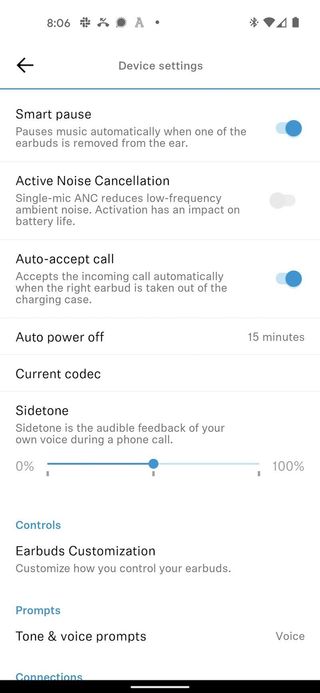The image displays a cell phone screen featuring multiple settings and indicators. At the top left, the screen shows "806" and indicates a missed call and a new text message. An "A" icon and a dot are also visible. On the right side of the screen, there are icons for Bluetooth, Wi-Fi, cellular signal, and a fully charged battery. 

In the center, "Device Settings" is prominently displayed, followed by a left-facing arrow on the left side underneath a teal-blue line. Below this line is a list of various device settings.

- **Smart Pause:** This setting is toggled on, indicated by a blue switch. It describes functionality that automatically pauses music when one of the earbuds is removed from the ear.
- A thin light-gray line separates this from the next setting.
- **Active Noise Cancellation (ANC):** This setting is toggled off. It mentions that single mic ANC reduces low-frequency ambient noise and that activation impacts battery life.
- Another dividing line follows.
- **Auto Accept Call:** This feature is enabled, indicated by a blue toggle. It automatically accepts incoming calls when the right earbud is removed from the charging case.
- Yet another dividing line precedes the next setting.
- **Auto Power Off:** This setting is configured for 15 minutes.
- **Current Codec:** This section is labeled "C-O-D-E-C."
- **Slide Tone:** An option allows the user to adjust the audible feedback of their own voice during a phone call. The setting ranges from 0 to 100, and the current level is set in the middle, indicated by a blue slider bar.

At the bottom of the screen, "Controls" is highlighted in blue, pointing to additional adjustable features.